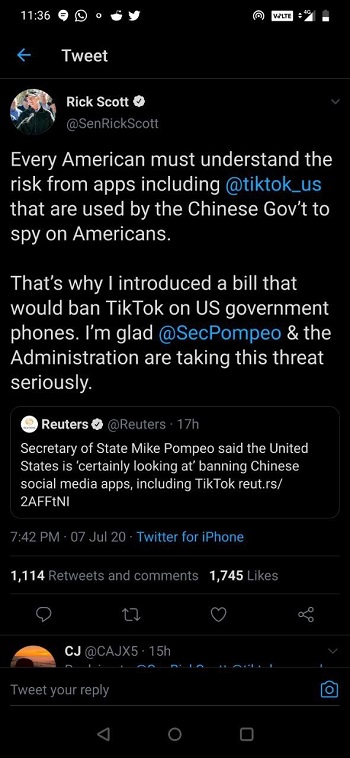This image is a screenshot taken on a smartphone, evidenced by the time, battery percentage, reception information, and various notifications displayed at the top of the screen. The screenshot captures the Twitter app in dark mode, where the background is entirely black, and text is primarily white, with links highlighted in blue and auxiliary details in gray.

The focal point of the screenshot is a tweet from a verified user named Rick Scott, who is presumably a senator. The tweet comprises a critical message regarding the risks posed by apps like TikTok, which Senator Scott claims are used by the Chinese government for spying on Americans. He mentions introducing a bill to ban TikTok on U.S. government phones and expresses approval of the administration and Secretary of State Mike Pompeo's actions in addressing this concern.

Senator Rick Scott's tweet is a direct response to a tweet from Reuters posted about 17 hours earlier. His tweet was made on July 7, 2020, at 7:42 PM from an iPhone. The screenshot also shows the engagement metrics for the tweet, including the number of likes, retweets, and comments.